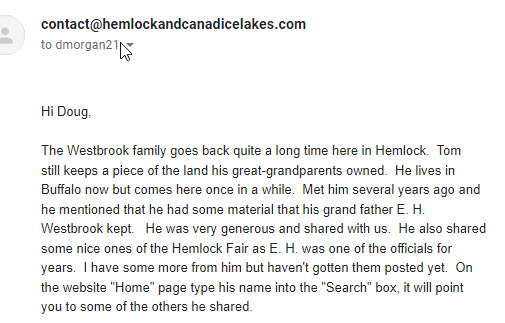This image is a screenshot of an email displayed on a computer. The email, set in black text on a white background, is addressed to DMorgan21 and is from contact@hemlockandcandislakes.com. The email begins with a greeting, "Hi Doug," and goes on to talk about the Westbrook family, who have a long history in Hemlock. Tom Westbrook, who resides in Buffalo but occasionally visits Hemlock, still retains a piece of land that belonged to his great-grandparents. The email mentions that several years ago, Tom shared some material kept by his grandfather, E.H. Westbrook, who was a long-time official at the Hemlock Fair. Although some of this material has not yet been posted, the email advises that entering E.H. Westbrook's name into the website’s search box will lead to other shared items. The general layout includes the email text centered within the image, framed by the conventional email interface in shades of white, black, and gray.